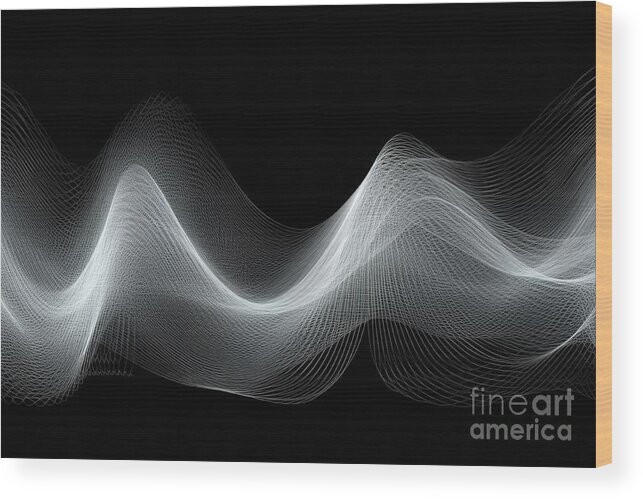The black and white image titled "Fine Art America" showcases a finely detailed piece of line art on a canvas that appears to be mounted on a wooden frame. The artwork features multiple undulating lines, resembling an EKG heartbeat or a wave pattern, which collectively form a layered, woven texture. The lines are predominantly white, becoming more intense and brighter in the center and gradually fading to gray towards the edges. This is set against a black background speckled with subtle gray swirls, enhancing the three-dimensional illusion of the piece. The artwork seems tilted, giving it a 3D perspective, further accentuated by the visible wood grain on the right side, highlighting its canvas on wood presentation. The raw, light tan wood frame contrasts with the sophisticated art, grounding the entire piece, which bears the signature "Fine Art America" in white text at the bottom right corner.